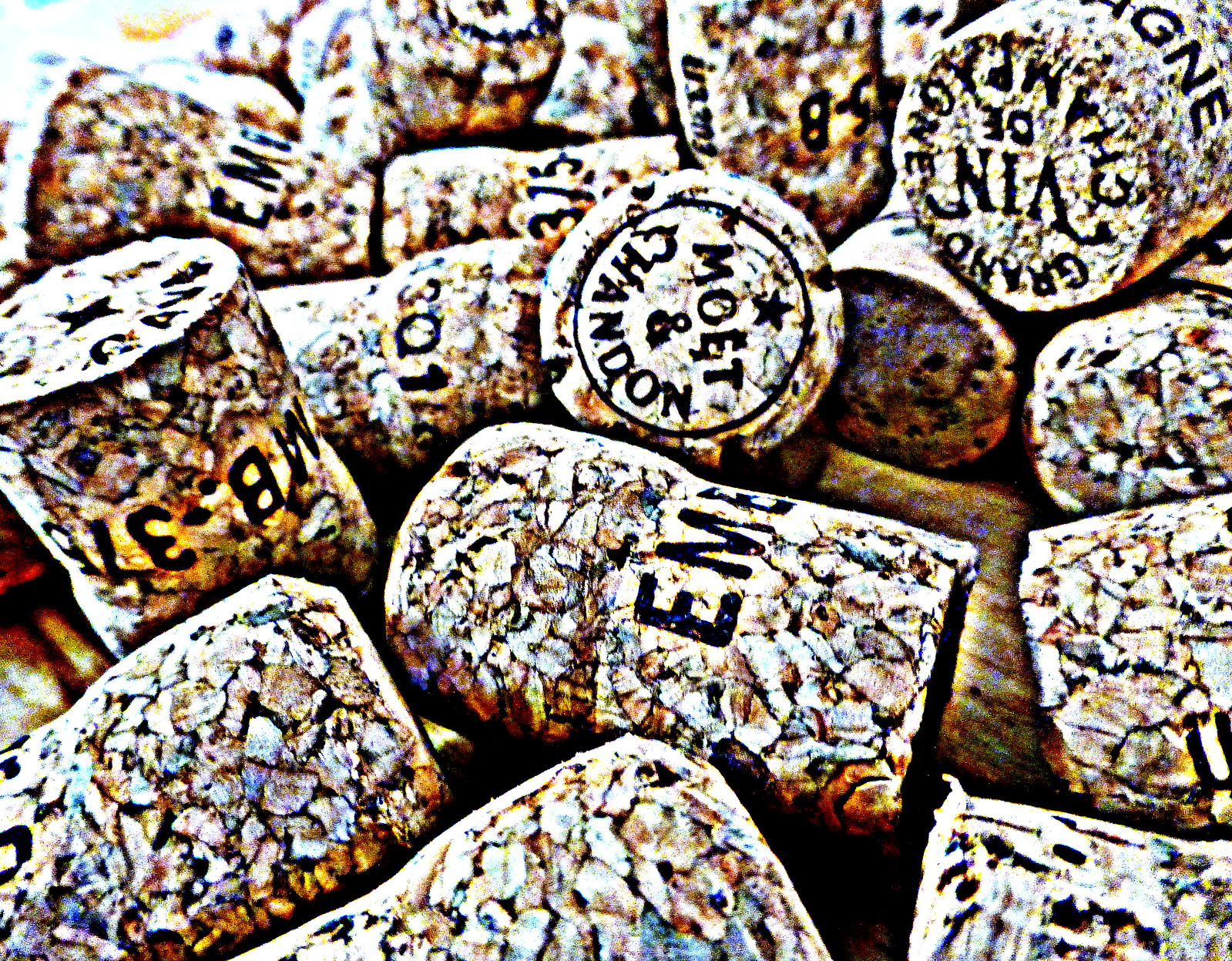The image is a large, somewhat blurry photograph, especially in the upper left-hand corner, of numerous champagne corks stacked and scattered in various directions. The corks are brown and white with a speckled appearance and small cracks throughout. Prominently featured in the center is a cork with the inscription "Moet & Chandon," complete with a star above the text. Another cork in the middle lies on its side and bears the letters "E-M-E" in bold, black all-caps. There's also a visible inscription on a cork in the upper right corner mentioning "champagne." The image appears to have a glossy, rainbow-like sheen, suggesting it may have undergone a computerized filter. Though there are no mugs or jars, the filter's visual distortion adds a unique, almost patterned texture to the corks.